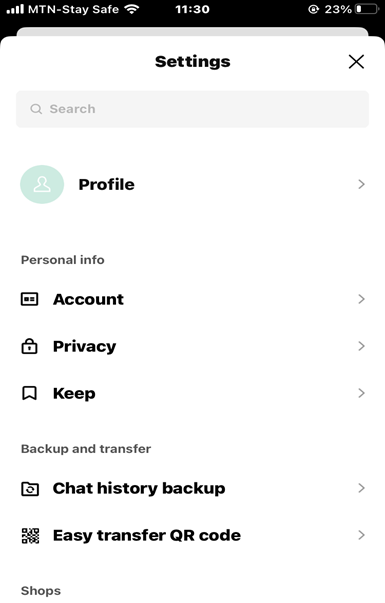This image is a detailed screenshot taken from a mobile device. At the top of the screen, there is a black header featuring several icons in white, including network connection (identified as "MTN stay safe"), Wi-Fi signal strength, the current time, and battery status.

The main part of the screenshot shows a white background, overlaid by a pop-up settings menu that occupies the entire screen. At the top of this menu, the title "Settings" is displayed in bold black text. Directly beneath this, there is a grey search bar with the placeholder text "Search."

An icon of a profile is featured prominently just below the search bar. This icon is circular, green, and contains a simple white silhouette of a person. Underneath this profile icon, there are three labeled options under the section "Personal Info": "Account," "Privacy," and "Keep," each accompanied by a right-facing grey arrow indicating that there are additional options to explore.

Further down, the "Backup and Transfer" section is present, offering functionalities such as backing up chat history or performing an easy transfer via a QR code. Similar to the previous options, each item in this section also features a right-facing grey arrow for further navigation.